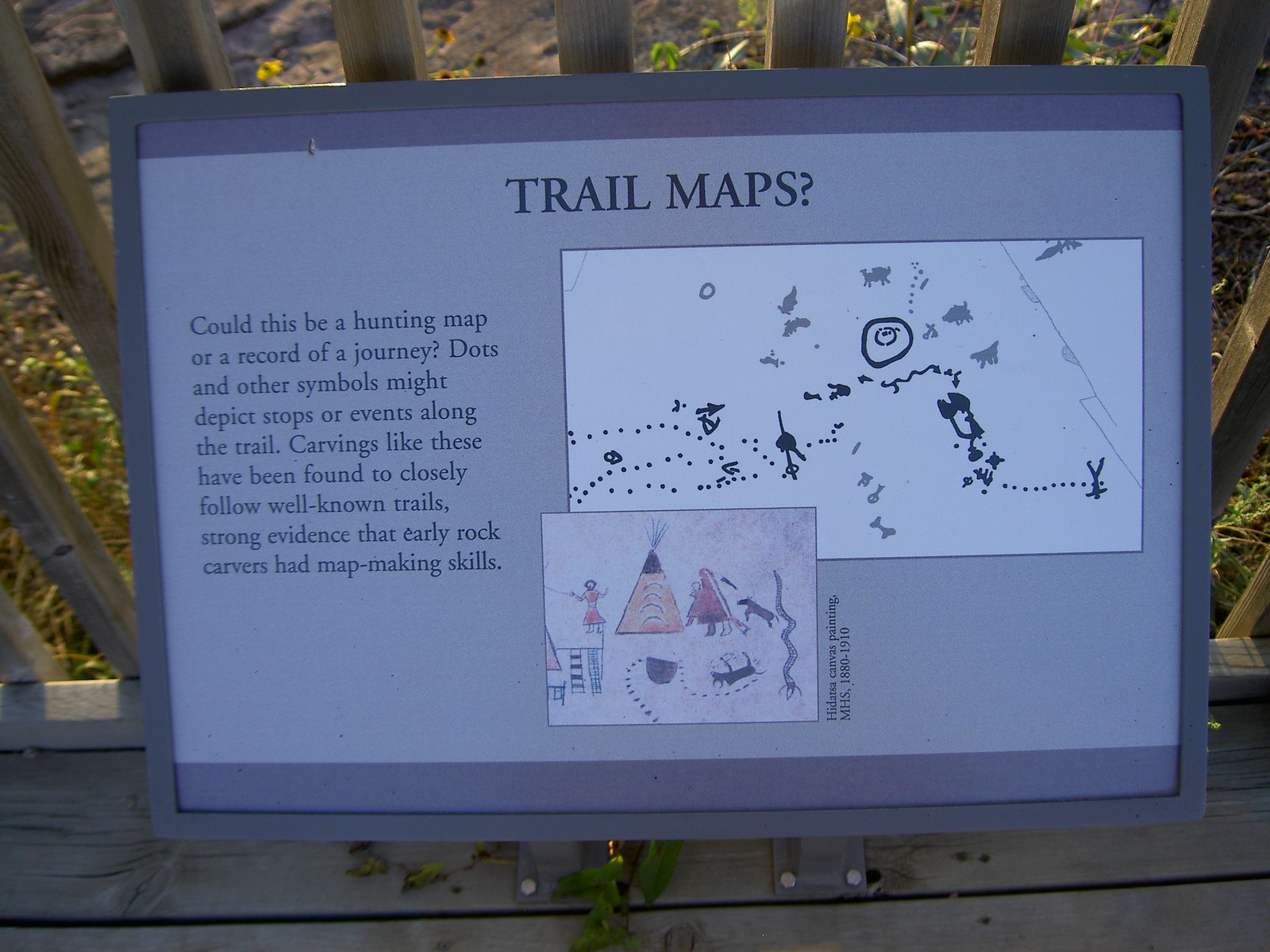An outdoor trail map is displayed on a plaque, framed in metal, and bolted to a wooden deck with a guardrail, overlooking a shrub-surrounded cliff. The map has a lavender background and features the words "Trail Maps?" in large text at the top. To the right, it presents a low-detail, black and white hunting map with dots indicating stops or events along a trail. On the left, a paragraph questions whether the map records a journey or hunting activities, suggesting strong evidence that early rock carvers possessed map-making skills. Below, a small, older map and Indian depictions of life show a teepee, animals, and people. A small diagram to the side highlights places where such carvings have been found, along with a photo captioned "Hidatsa canvas painting, MHS 1880 to 1910."